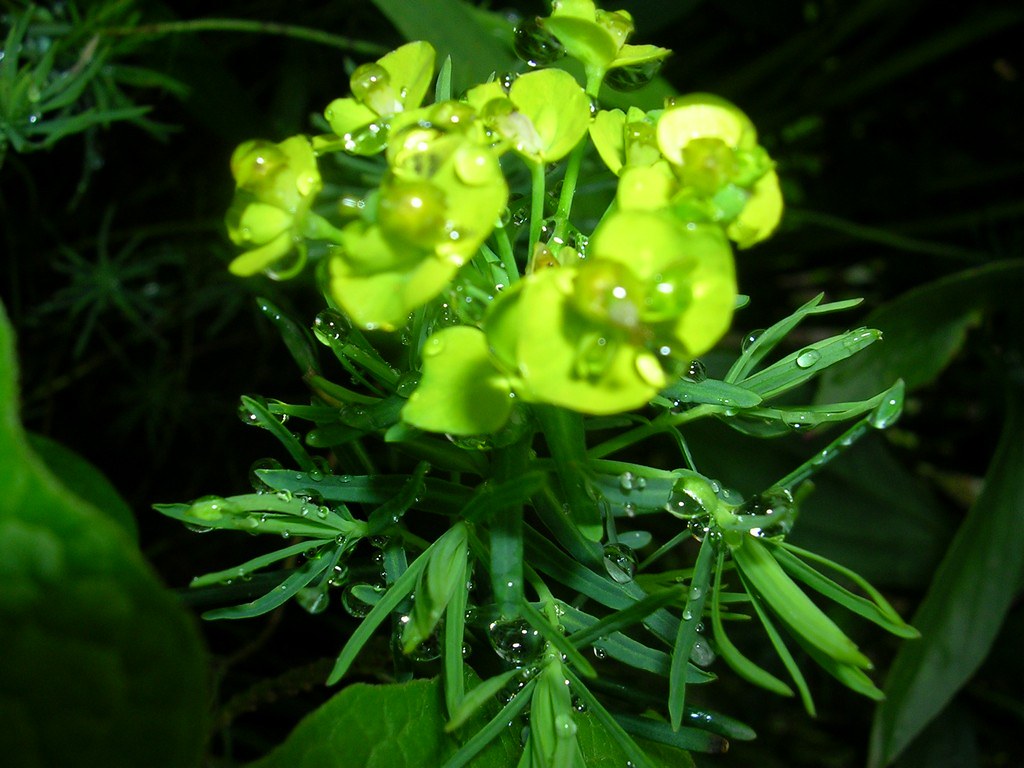The photo captures a highly detailed and vivid image of a green plant, likely taken outdoors, that glistens with numerous water droplets, indicative of a recent rain or watering. The plant’s leaves are slender and quite fine, resembling the spiny leaves of rosemary herbs. As one's eye moves up the plant, the color transitions to a brighter, almost lime green at the top, where the leaves appear to sprout similarly to a bulb. Natural light illuminates the topmost part of the plant, highlighting some bulbous, marble-like formations in the center of the blooming flowers, faintly reminiscent of pacifiers. The base of the plant is set against dark soil, possibly in a pot or planter, with shorter, vine-like neighboring plants sprawling out in different directions, adding to the intricate organic scene.